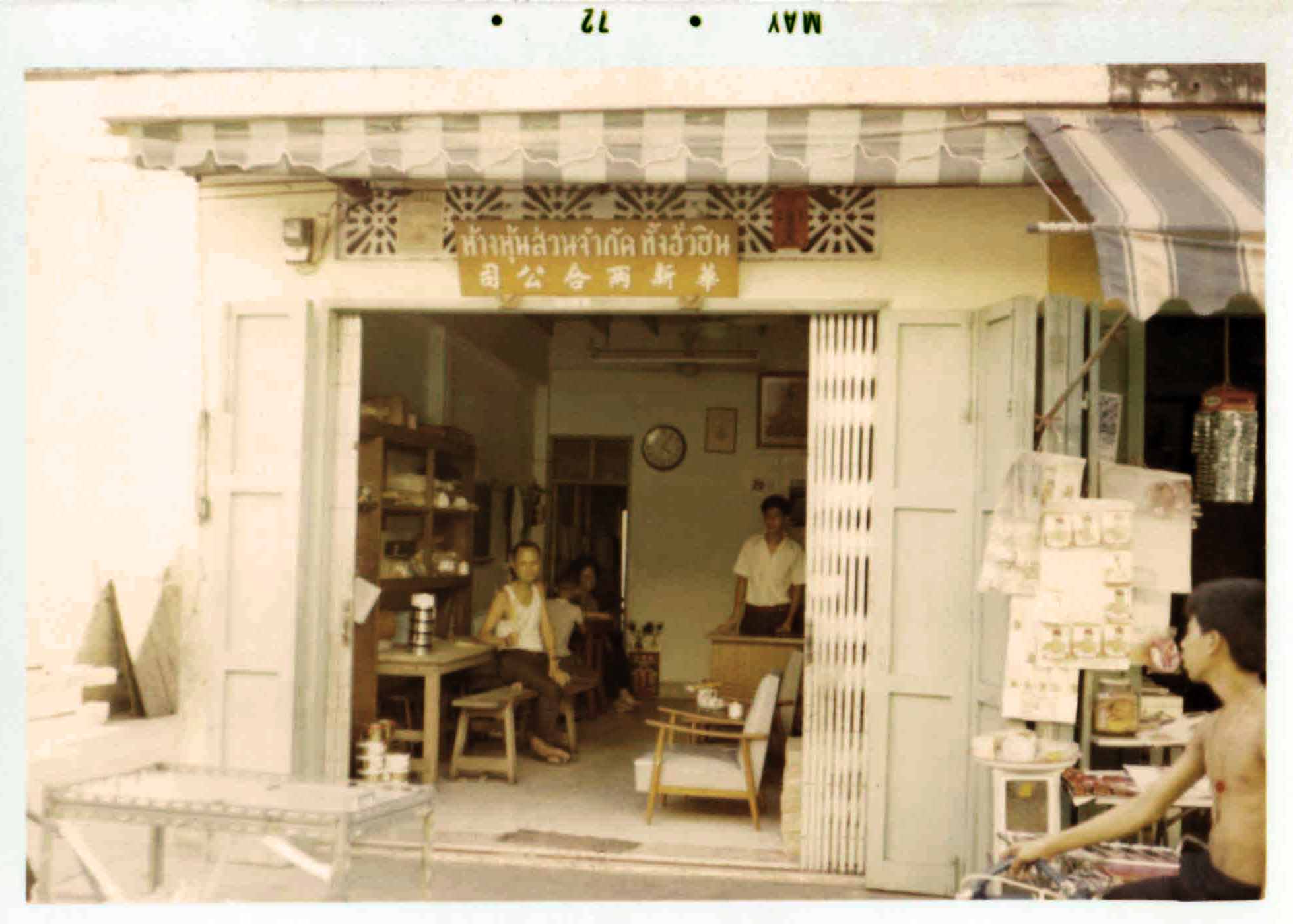In this daytime outdoor image, we observe an open, whitish building that could be a garage or living space, featuring an inviting open door. Inside, the focal point is a man dressed in a white tank top, lounging on a bench with his elbow resting on a table. In front of him sits a young woman, possibly his wife, cross-legged on the same bench. Their young boy stands behind her, while another man in a white shirt stands behind a counter or desk. A range of furniture populates the room, and a clock adorns the wall, along with a sign bearing foreign script. The scene extends outside the building, where a bare-chested teenage boy with dark hair rides a bicycle near the door's entrance, highlighting the carefree, familial atmosphere of the setting.